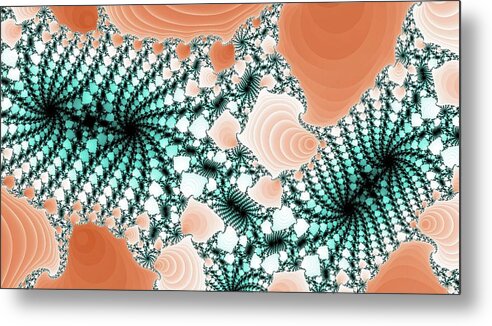This artistic rendering features a fractal-based design, characterized by four prominent spirals—two on each side—seamlessly blending black at the center into vibrant shades of green and turquoise. Surrounding these spirals are smaller, intricate swirls and circular formations that extend outward, creating a galaxy-like pattern. The background is a delicate mosaic of light pink and salmon hues, reminiscent of uncooked chicken breast, interspersed with globs of the same pink that resemble seashells. Additional splashes of orange and creamy white accentuate the spirals and circles, creating a unique, dynamic, and colorful visual experience. This digital artwork is framed by a subtle, small black border, completing its distinctive, ethereal appearance.